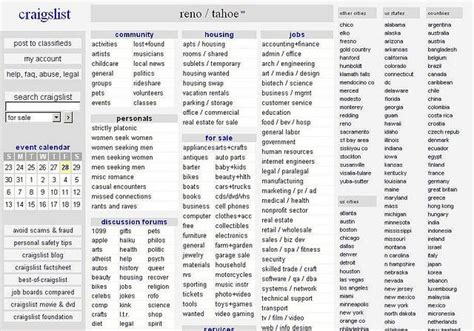This image is a screenshot of the Craigslist website for the Reno/Tahoe region. Centered on a wide, white background, the page displays the Craigslist logo prominently in the upper left corner, accompanied by a vertical navigation menu. This menu contains several clickable buttons: "post to classifieds," "my account," "help, FAQ," and "abuse, illegal." Below these, a search bar allows users to "search Craigslist," defaulting currently to the "for sale" section.

Continuing down the left side, an event calendar is visible, along with several essential links such as "avoid scams," "safety tips," "blog," and "facts." Taking up the majority of the right side, multiple columns categorize the main content areas of the site. These headers include "community," "personals," "discussion forums," "housing," "for sale," and "jobs." Additionally, an "international" section is situated to the far right.

At the bottom of the screenshot, the content seems truncated, possibly cutting off a calendar or other feature. The image resolution is notably small, making finer details hard to discern. Overall, the layout is minimalist, utilizing simple text links and some light gray panels to delineate sections such as "community" and "personals," adhering to Craigslist's customary sparse design.